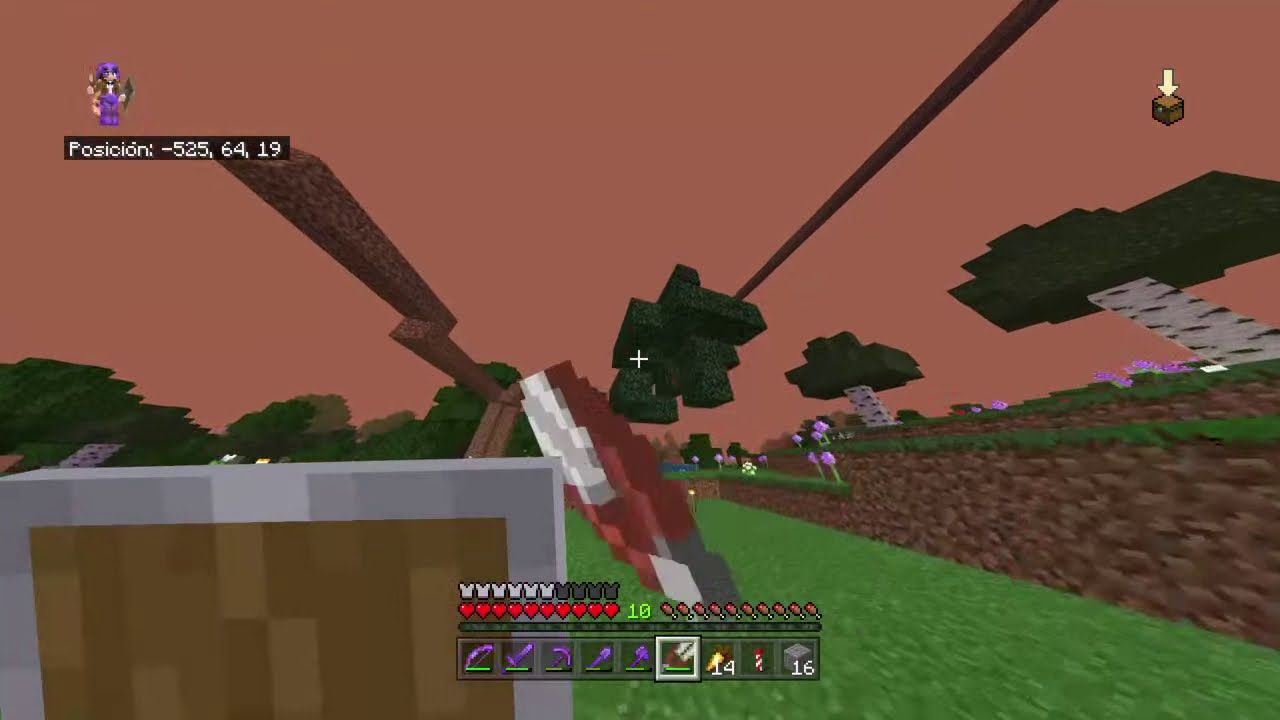This is a screenshot from a block-building video game, likely Minecraft, featuring a pixelated, pinkish-brownish-red sky in the background. The foreground is populated with various game icons and elements, including heart icons with a green number "10", indicating health, and two sets of purple objects that resemble weapons, numbered "14" and "16". A brown box with a silver trim is visible on the left. The character’s coordinates, displayed at the top left, read (-525, 64, 19). The right side showcases a tan-colored wall with a grassy top, leading to a background that includes green trees with white trunks. There is green grass at the bottom, and the middle of the image hints at a blurry, pixelated figure, possibly a character in a purple outfit. The bottom toolbar, which appears clickable, includes various game tools and options, enhancing the gameplay experience in this outdoor setting.